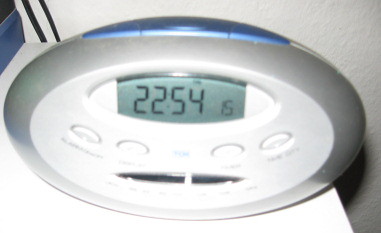A sleek, oval-shaped clock rests elegantly on a pristine white counter, set against a light gray background. The clock features a minimalist design with a white face, encircled by a subtle gray frame. At the top, three buttons in a light blue, almost turquoise hue, add a touch of modern sophistication. The digital display on the clock shows the numbers 22, 54, and 15, indicating the current time in an orderly fashion. This clock seamlessly combines functionality with contemporary style, making it a chic addition to any setting.